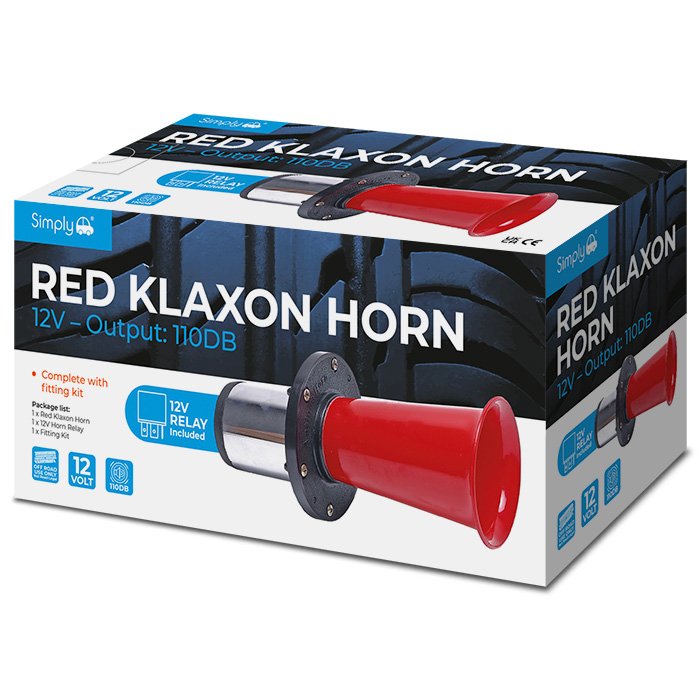This image depicts a box containing a red klaxon horn, set against an all-white background. The front of the box, along with the right-hand side and the top, share identical designs featuring a combination of navy at the top and white at the bottom, accented with turquoise labels. The upper half showcases a blue area where, in white text, it reads "Red Klaxon Horn," followed by specifications "12-volt output, 110 dB" in blue. The lower half of the box displays a picture of the horn itself, which features a shiny red horn cone attached to a black disc with a chrome metal handle in the back. Also shown is the Simply brand logo, comprising a simplistic white car resembling a ladybug car. Additional text on the box states, "Complete with Fitting Kit," along with a package list detailing the contents: 1 Red Klaxon Horn, 1 12-volt horn relay, and 1 Fitting Kit.